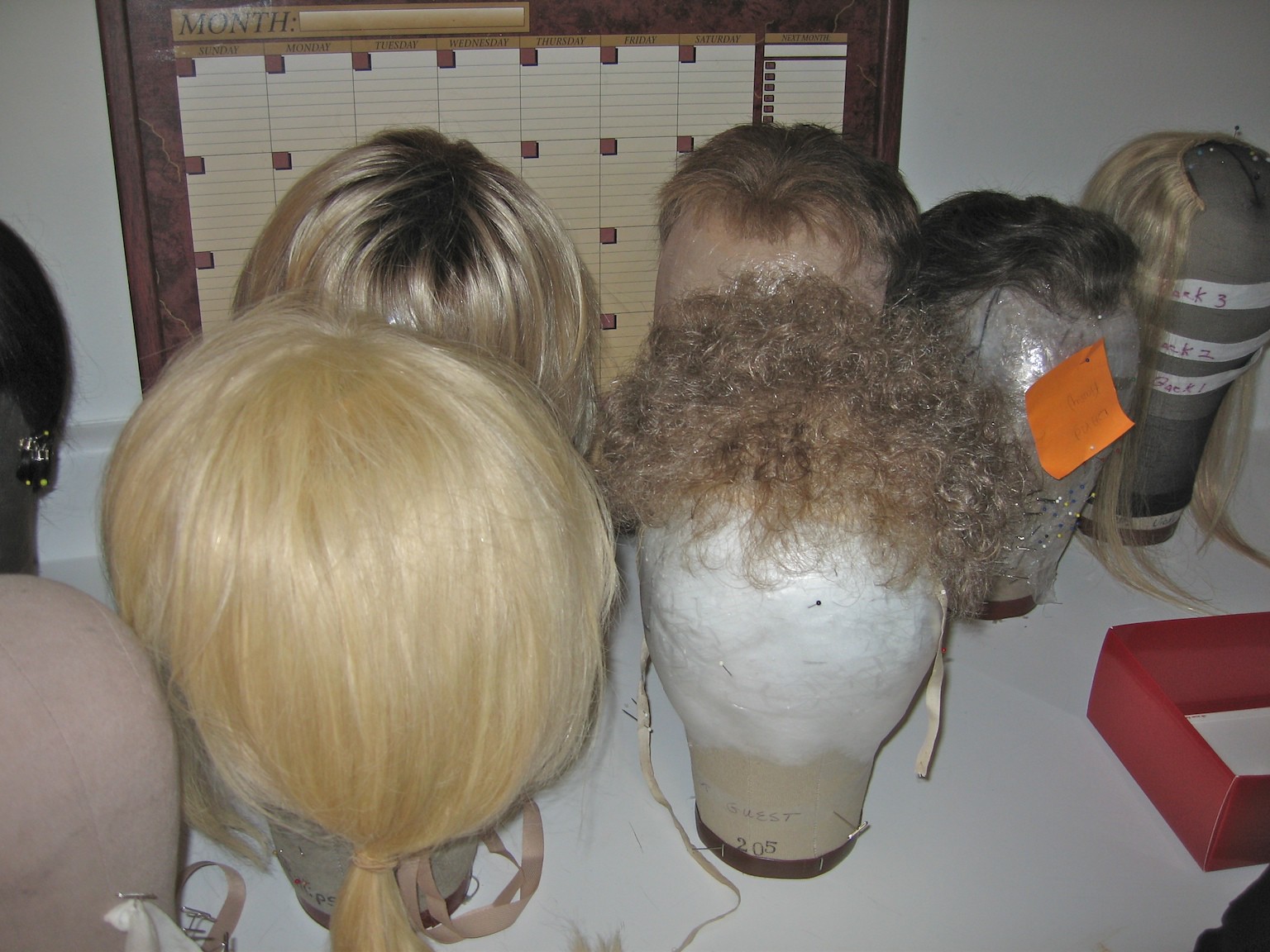This photograph captures an indoor scene where eight styrofoam mannequin heads are displayed on a white Formica counter. Each head, devoid of facial features, serves as a holder for a variety of wigs, showcasing an array of hairstyles and colors. From left to right, there is a very light blonde ponytail wig, a short curly brownish-gray wig, a short, cropped men's wig, a wavy men's wig, and a straight blonde wig with no bangs. Other wigs include a short wavy brown hairdo and straight blonde hair. The dimly lit environment suggests the use of a flashlight or camera flash as the main source of light. Various wigs indicate a display of hairpieces that could be for men or women, likely intended for theatrical use or showcasing craftsmanship. In the background, a reusable dry-erase calendar is mounted on the wall. Some of the mannequin heads feature additional accessories like post-it notes or tape, adding distinguishing features to the otherwise blank faces.